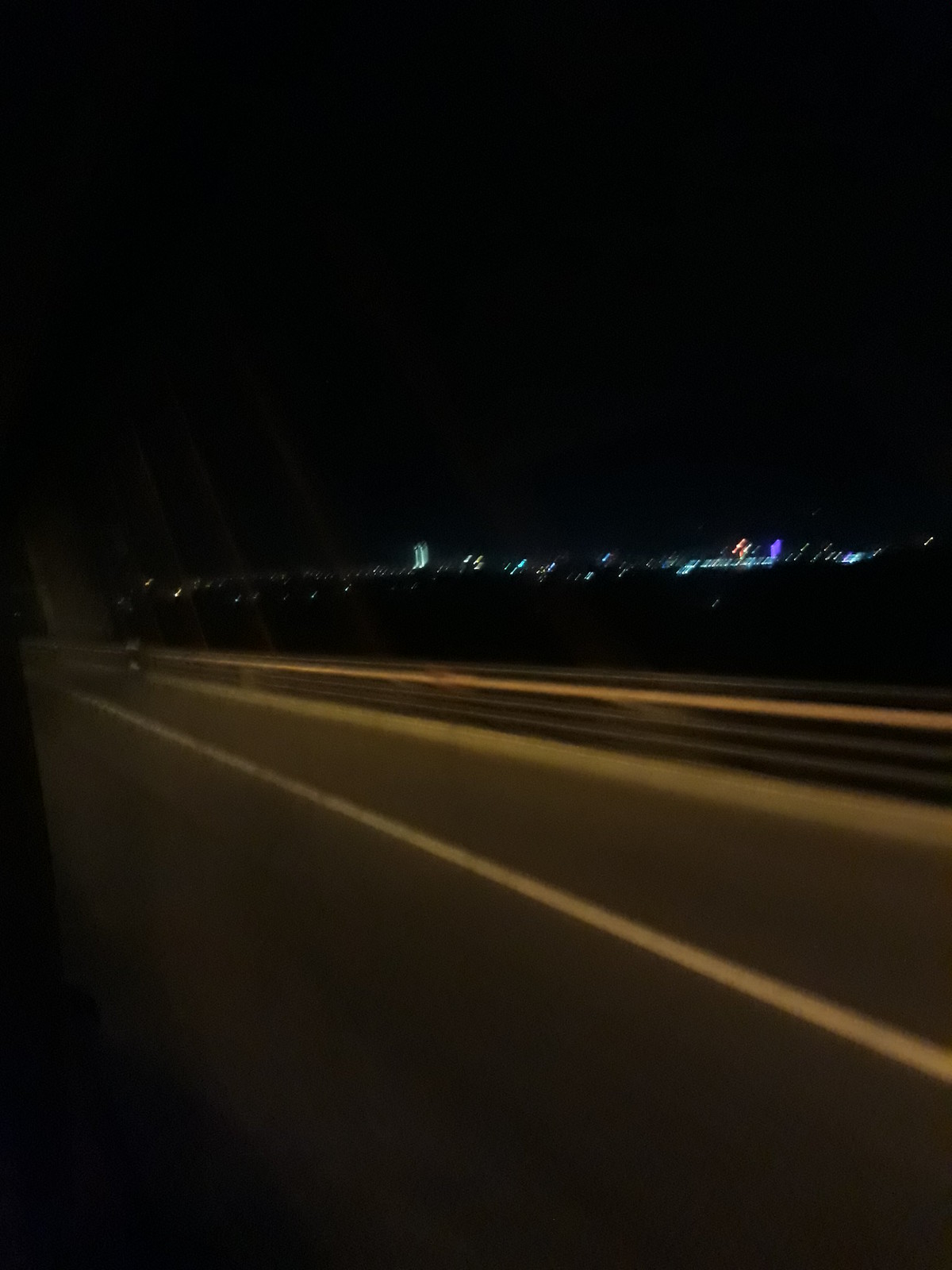The image captures a nighttime scene viewed from the passenger seat of a vehicle traveling along a highway. The scene features the right side of the highway characterized by a stark gray surface and a prominent white vertical line marking the outer edge of the lane. A protective railing runs along the side, suggesting the highway may be elevated, possibly over a bridge. In the distance, the horizon fades into a deep black, punctuated by a sparse array of tiny, glimmering lights that signal a distant cityscape. The city lights, though minimal, highlight the silhouette of a few structures. Above this faint urban glow, the sky stretches across the entire frame in a vast, uninterrupted expanse of darkness, amplifying the serene isolation of the highway at night.